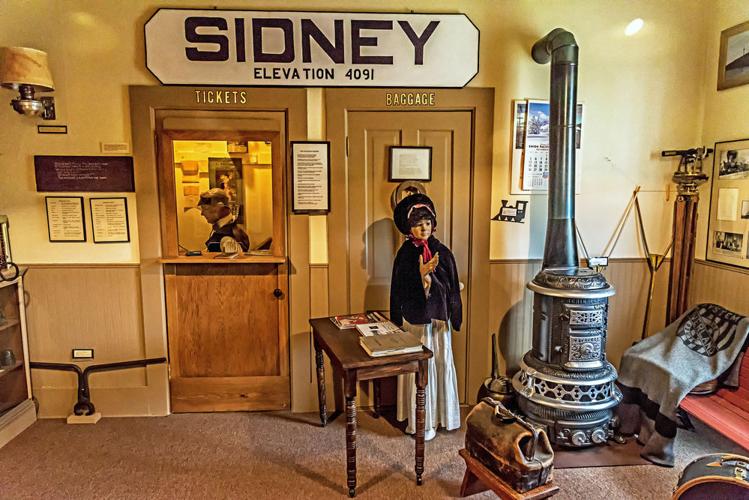The image is a detailed representation of an old-fashioned ticket counter, possibly from a model of a train station or transportation office in Sydney. It's a rectangular photograph showcasing a miniature diorama. The centerpiece is a prominent white sign at the top center-left that reads "SYDNEY" in large, all-caps letters, with "Elevation 4091" right below it.

Beneath the sign are two wooden doors, both framed in black. The left door labeled "Tickets" features a square cut-out in its upper portion, through which a tiny, detailed figure resembling a person can be seen. This figure could be a woman or a man, wearing what appears to be a black cap and engaged in some activity at the counter.

The right door, marked "Baggage," stands closed. In front of it is a doll-like figure of a woman dressed in a black top, long light-colored skirt, and black bonnet, with dark hair. She is positioned near an old metal stove, whose pipe extends into the back wall. The walls of the room are yellow at the top and brown wood at the bottom, creating a warm, vintage atmosphere.

In the upper left corner of the image, there is a small wall-mounted lamp. A calendar is partially visible behind the stove's pipe. Additionally, a wooden table with four legs extends towards the viewer, situated to the left of the woman standing by the baggage door. This table has two books resting on it. The floor is covered in brown carpeting, adding to the antiquated aesthetic of the scene.

This meticulously crafted model provides a nostalgic glimpse into a bygone era, filled with carefully placed miniature items and figures that enrich the overall narrative of the setting.